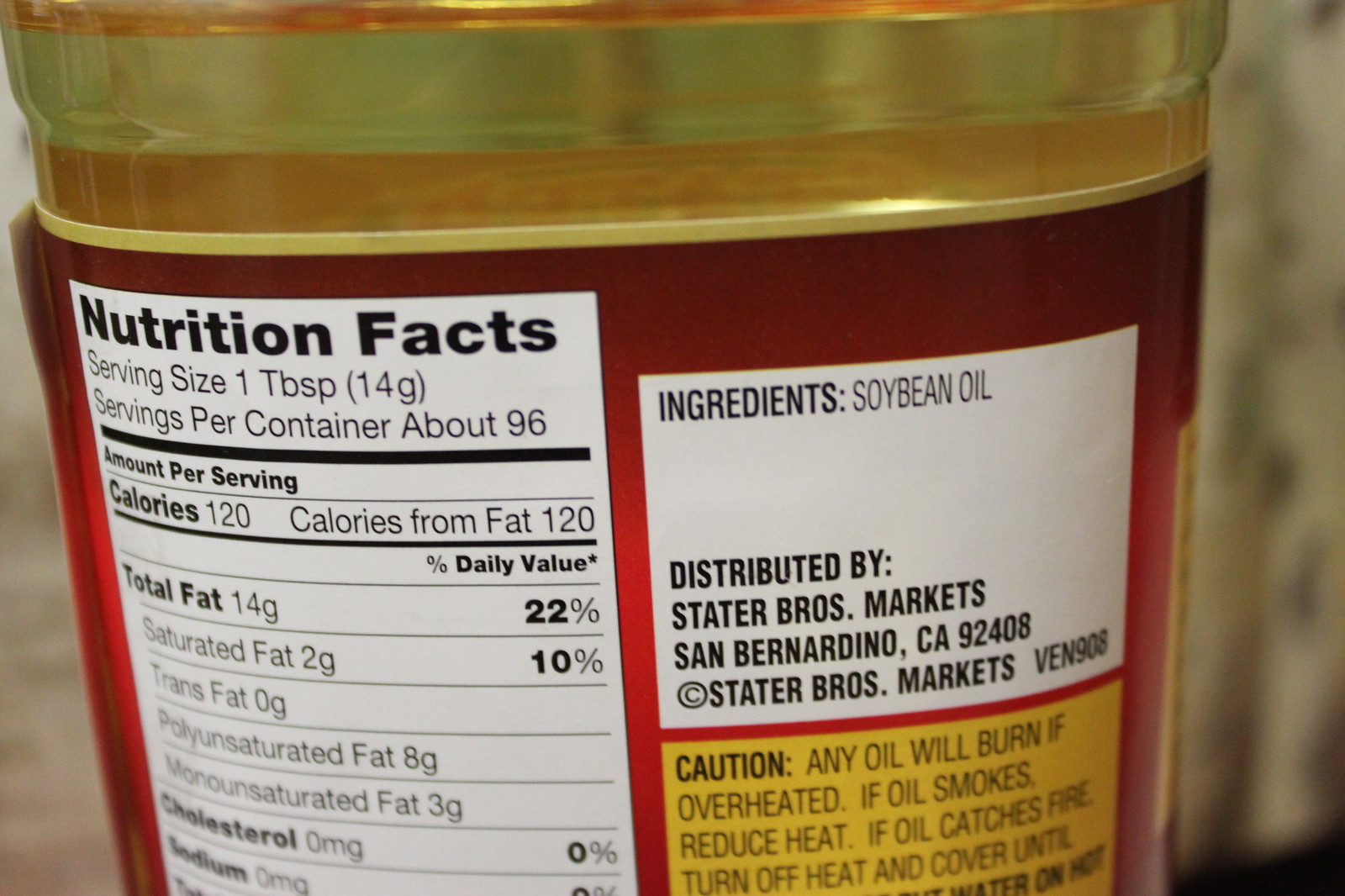The image showcases the nutrition facts and ingredient list of a food product, likely contained in a glass jar. The focus is primarily on the text, making identifying the exact product difficult. The visible part of the packaging appears to be glass, hinting it might be soybean oil. 

The ingredients list confirms soybean oil, and the product is distributed by Stater Bros. Markets, San Bernardino, California, 92408. The label also features a cautionary note about the oil's flammability, advising to reduce heat if the oil smokes and to turn off heat and cover if it catches fire, though part of the warning text is cut off.

On the left side, the nutrition facts are displayed, with the following details:
- Serving Size: 1 tablespoon
- Calories: 120 (all from fat)
- Total Fat: 14 grams (22% of the daily value)
- Saturated Fat: 2 grams (10% of the daily value)
- Cholesterol: 0 mg
- Sodium: 0 mg

The background of the image is blurry, showing a grayish object that is not discernible.